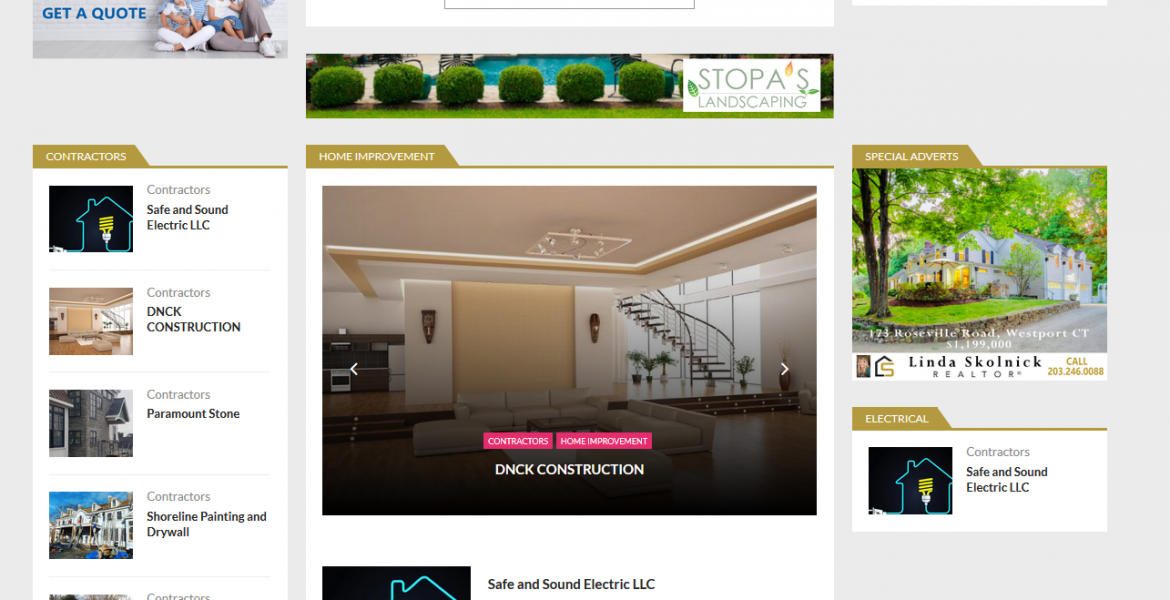**Website Overview of Stapa's Landscaping**

The image features the homepage of Stapa's Landscaping, set against a shaded background with a prominent display of expertly sculpted green bushes. 

**Header Section:**
- On the right is a white square with the company name, "Stapa's Landscaping," elegantly inscribed in gray font.
- In the top left corner, a blue button reads "Get a Quote."

**Family Imagery:**
- The upper section shows a partial image of a man and woman holding two children, although their heads are cropped out of the frame.

**Contractors Listings:**
- Below the "Get a Quote" button, the word "contractors" appears in white against a light brown banner.
  - Listed are:
    - **Safe and Sound Electric, LLC**
    - **DNCK Construction**
    - **Paramount Stone**
    - **Shoreline Painting and Drywall**

Each contractor listing is paired with an image on the left side.

**Stapa's Landscaping Banner:**
- Underneath, a brown banner with white text reads "Home Improvement."
- It features a home interior with a visible staircase, accompanied by another banner stating "contractors" in white on a pink background.
- Another pink banner highlights "Home Improvement," followed by the company name "DNCK Construction" in white.
- Below the image, the text "Safe and Sound Electric, LLC" is also mentioned, but partially cut off.

**Special Adverts Section:**
- On the right side, against a brown banner, the term "Special Adverts" appears.
- Featured is a picturesque white house with illuminated windows and well-maintained landscaping.
- Below, the Realtor's information is provided:
  - **Linda Skolnick, Realtor**
  - Call **201-246-0088**
  - Address: Westport, Connecticut
  - Price: **$1,199,000**

**Electrical Contractors:**
- Under Linda Skolnick's details, a brown banner labeled "Electrical" is displayed.
- Underneath, "Contractors, Safe and Sound Electric, LLC" appears, though it is partially cut off.